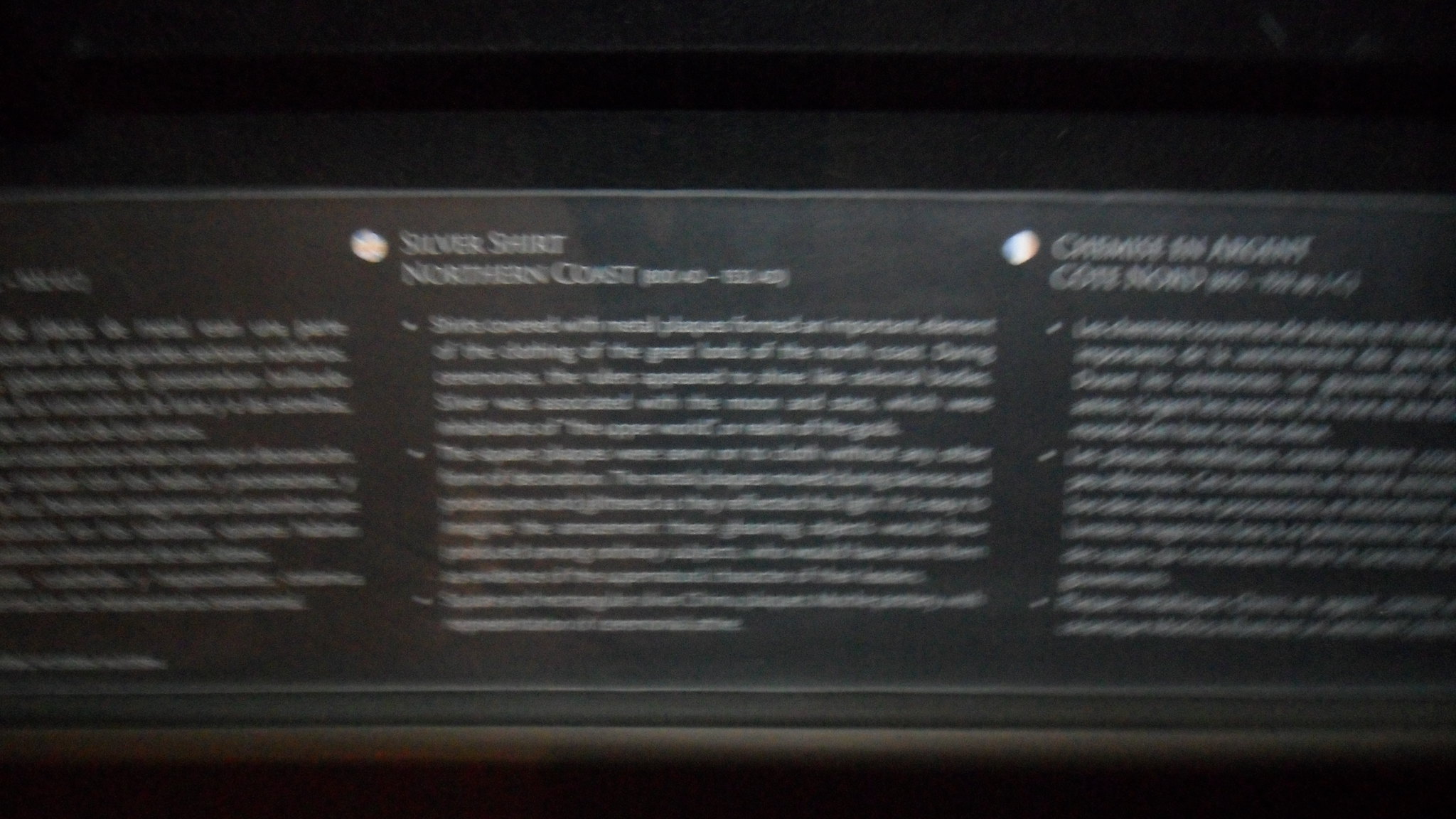In this horizontal photograph, a very blurry sign spans from left to right against a black background. The sign features three paragraphs of text, all rendered in white. Each paragraph is topped by a heading, which is partially legible despite the overall blurriness. The heading of the left paragraph is almost entirely cut off, leaving only one indistinct and unreadable word visible. The middle paragraph's heading reads "silver shirt, northern coast," but its remaining text is too blurry to decipher. The right paragraph follows the same fate as the left, with an illegible heading and indistinguishable content. Each paragraph is accompanied by three bullet points, though their content remains unreadable due to the blurred nature of the image.